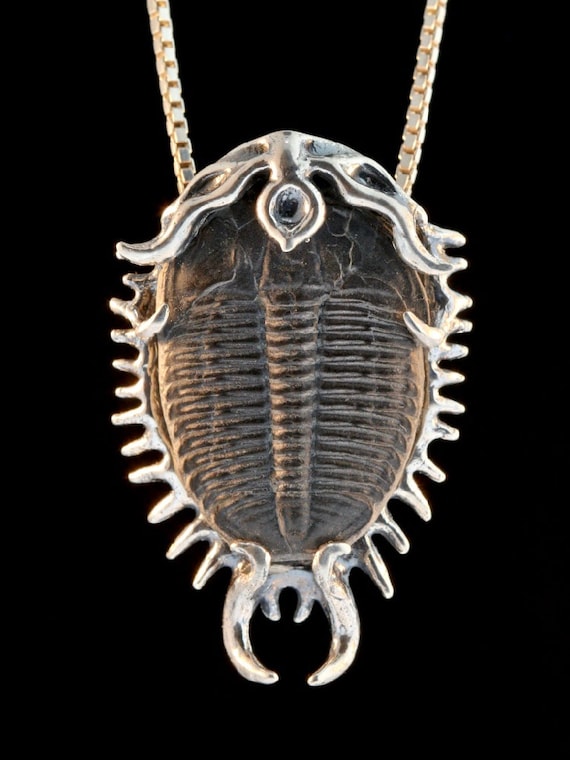This image showcases an intricately designed necklace, featuring a pendant that integrates a black, fossilized trilobite into its design. The fossil is encased in polished silver or pewter metal, which is shaped to resemble the structure of the trilobite. The pendant, which hangs from a silver chain, reveals detailed features such as a spiky outer edge and distinctive appendages, including two prominent points at the tail flanked by two smaller ones. Near the head, there is a circular jewel-like element, adding a touch of sophistication to the piece. The background is entirely black, emphasizing the pendant's metallic shine and the fossil's charcoal hue. While the metalwork appears polished, it bears some scuff marks, giving it a unique, hand-crafted character.